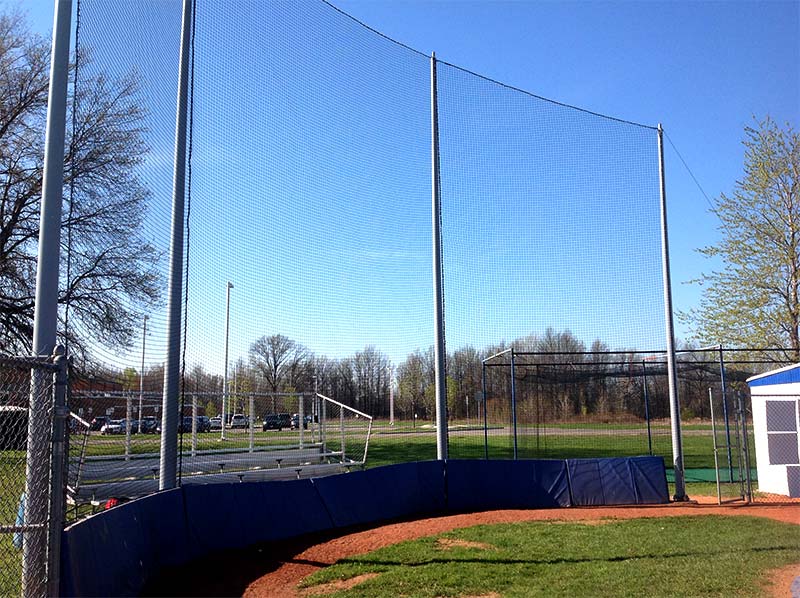The photograph captures a vibrant, modern baseball diamond under a bright blue sky with minimal clouds. A vast protective net, supported by four metal or concrete poles, dominates the scene. Leaning against this net are several blue padded rectangles. Behind the net, there are white or silver metal bleachers with safety rails. Further right, a fully-enclosed batting cage with nets on a metal frame can be seen. To the right of this structure, there's a fence with an opening leading onto the baseball diamond. The red clay track surrounds a patch of grass within the field. In the background, park lights are visible, and trees with varying foliage frame the image—one bare on the left and one with green leaves on the right. Additionally, a white building with a blue roof, possibly a dugout, is visible on the right side of the image.